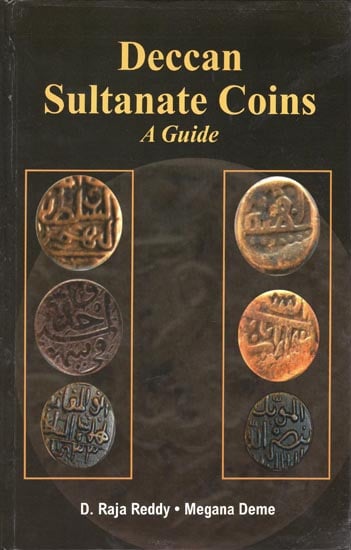The image depicts the front cover of a booklet against a dark background. The title "Deccan Sultanate Coins" is prominently displayed in gold-colored font at the top, followed by the subtitle "A Guide." The authors, D. Raja Reddy and Meghana Demi, are credited at the bottom in white text. Six ancient coins are arranged in two columns of three, each standing vertically. The coins vary in color, ranging from copper and bronze to shiny gold and dark black. Some coins are embossed with raised metal imprints, while others feature recessed designs. The inscriptions on the coins include Arabic text and possibly Egyptian-style symbols. Behind the coins, a large, faded bronze coin subtly emerges from the black background, enhancing the antique aesthetic of the cover.